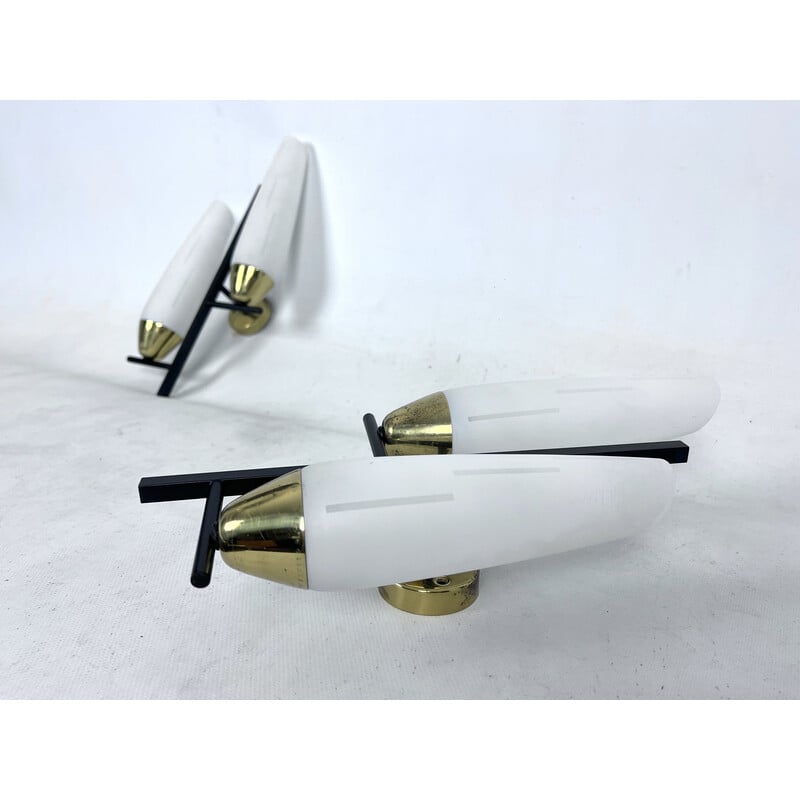In the image, there are two identical decorative objects that resemble rockets, each featuring an intricate design. Sitting on a curved surface in a white room, these objects include an elaborate gold top and a white, cone-shaped section at the bottom that narrows as it extends to the right. Both decorations are mounted on black handles connected to a brass base, which lies flush on the curved surface. The objects are positioned differently: one points upright from a dipped area and the other lies straight down over a flat part of the ground. The two sets of bars, one set lower and one set higher, extend horizontally from the central core of each object, which aids in balancing them within the room.